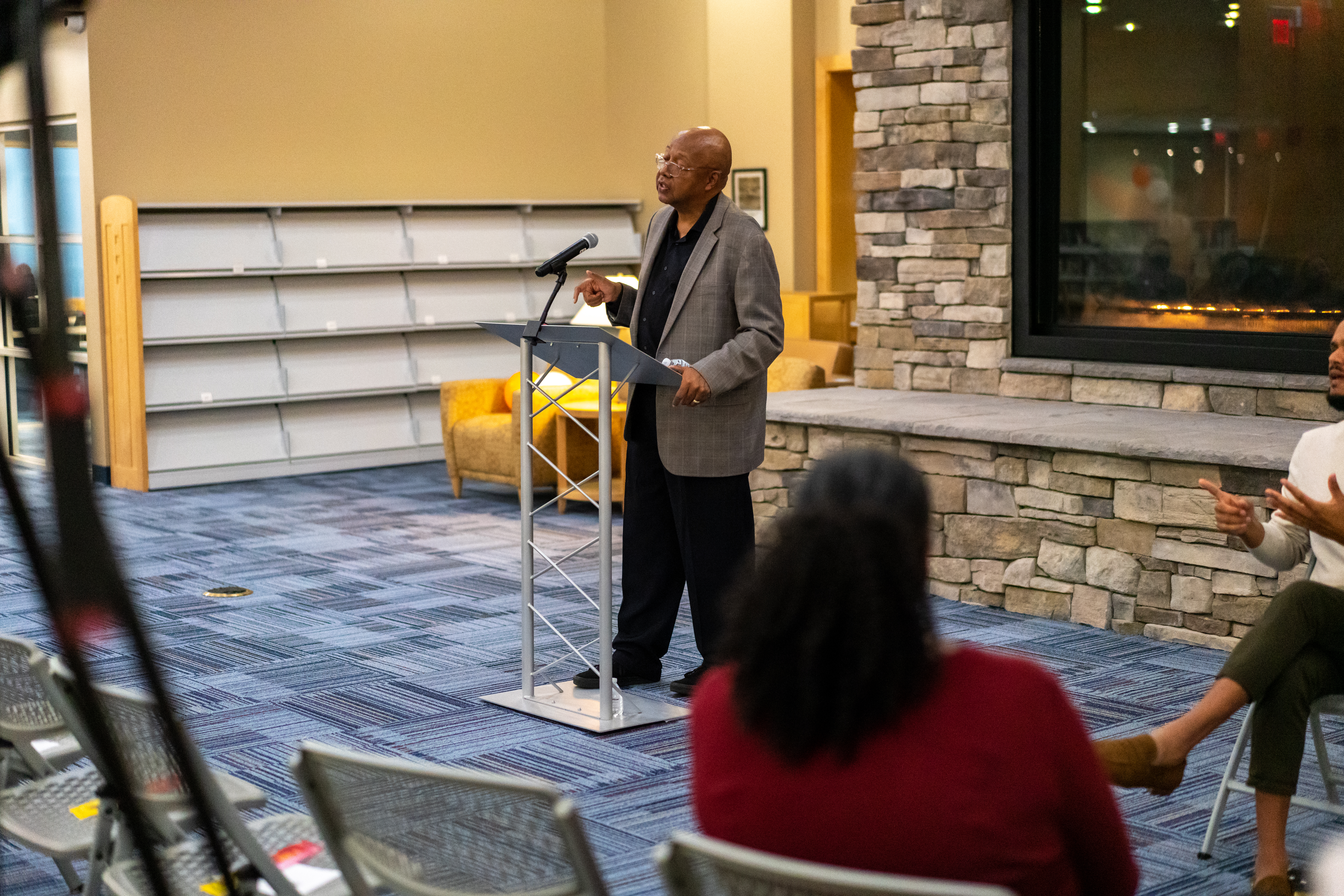In this detailed photograph, a distinguished man, who is likely a Harvard University professor of sociology, stands at a silver podium delivering a lecture. He is dressed in a gray collared jacket over a black V-neck shirt, paired with black slacks and shoes. The setting appears to be a well-lit, indoor space, possibly a library, suggested by the surrounding brick walls with glass panes in the middle and shelves to his left. The floor consists of a blue tiled pattern.

A woman, possibly serving as an interpreter using hand signals, stands to his bottom right, facing the audience, while another person is positioned to his right. The professor is actively gesturing with his right hand as he speaks. Behind him, a peculiar structure resembling a fireplace can be seen, adding an element of architectural interest to the scene. The audience is seated in front of him, attentively listening.

The background includes various shades of beige, orange, yellow, maroon, white, black, gold, gray, light blue, and dark blue, contributing to the photo's warm and dynamic color palette. The absence of text in the image directs focus towards the subjects and their environment. The scene exudes a scholarly atmosphere, with the professor looking towards the left side of the photo while the interpreter looks straight ahead.